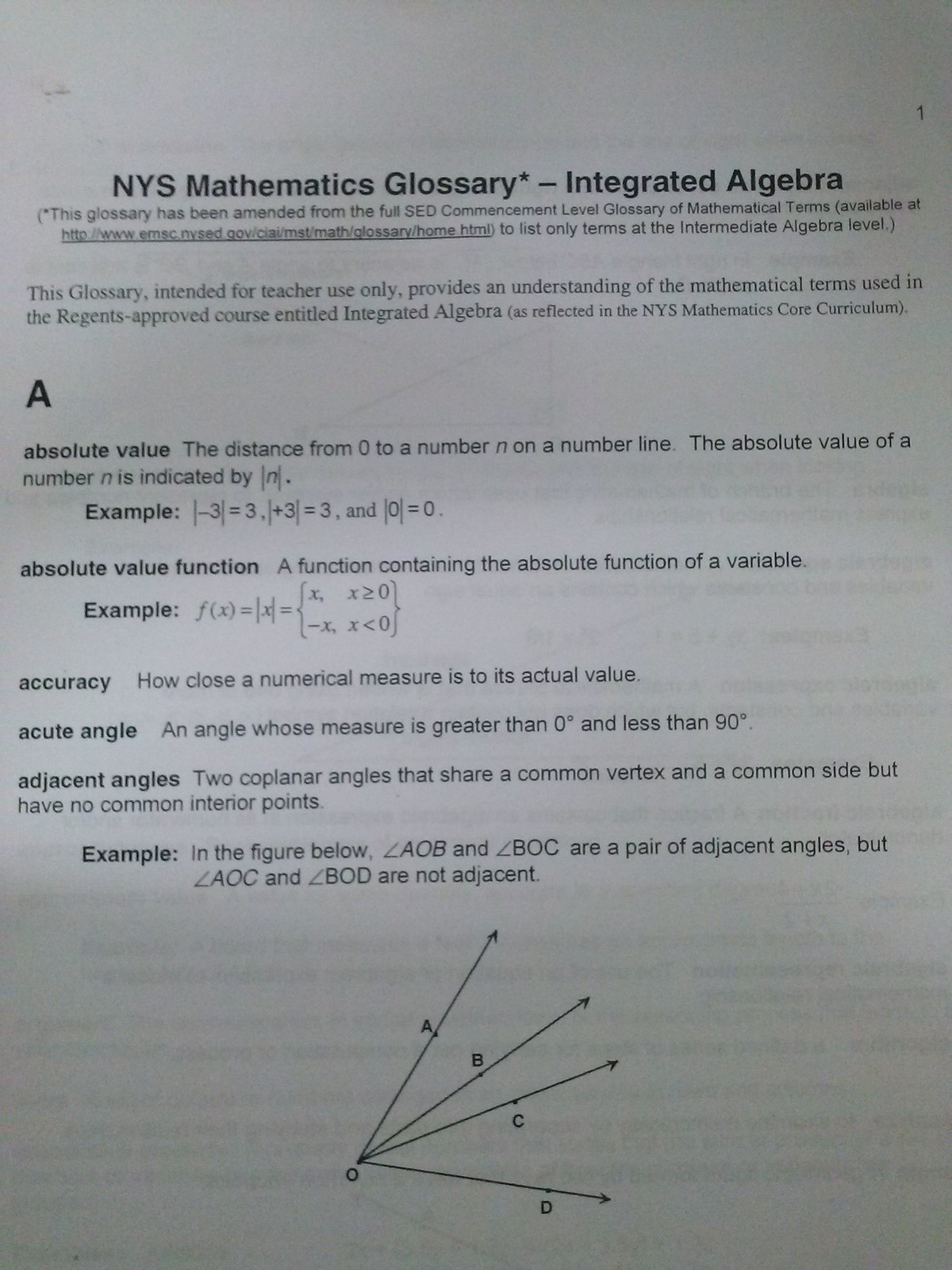The image depicts a portrait-mode photograph of a faded, grayish page from a mathematics textbook titled "NYS Mathematics Glossary - Integrated Algebra." The page is marked with the number one at the upper right corner, indicating it is the first page of the glossary. This glossary, intended for teacher use, provides definitions and examples of mathematical terms used in the Regents-approved course entitled Integrated Algebra, as reflected in the NYS Mathematics Core Curriculum. Starting with the letter 'A,' the glossary lists terms such as "absolute value," defined as the distance from zero to a number on a number line, followed by an example; "absolute value function," defined as a function containing the absolute value of a variable, with an example; "accuracy," described as how close a numerical measure is to its actual value; "acute angle," defined as an angle whose measure is greater than zero degrees and less than ninety degrees; and "adjacent angles," which are two coplanar angles sharing a common vertex and side but no common interior points, accompanied by an illustrative figure.